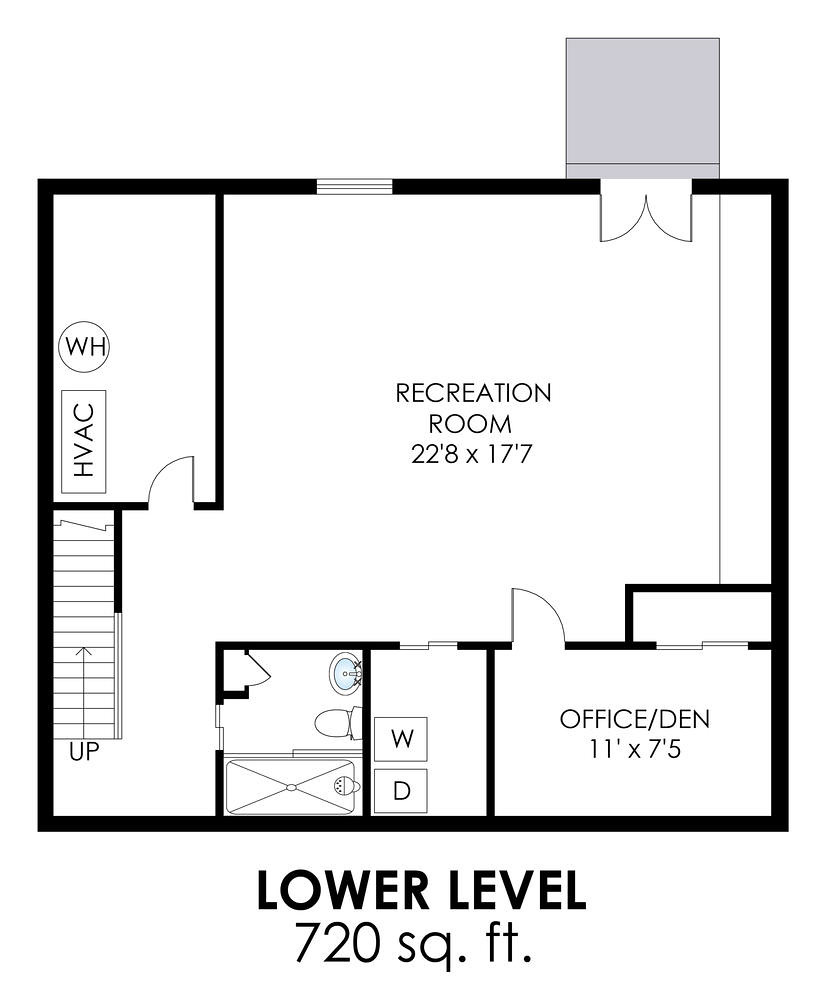This is a detailed floor plan of a lower level encompassing 720 square feet. The layout is square-shaped with distinct rooms and features. At the top right corner of the square, there is an attached gray square resembling an upside-down present, with what appears to be a bow area projecting into the main house. Centrally located at the top edge, a white line indicates a potential doorway.

In the upper left-hand corner is a smaller rectangular room marked "WH" (Water Heater) and "HVAC" (Heating, Ventilation, and Air Conditioning). Adjacent to this utility space is the largest room on the floor plan: the recreation room, measuring 22 feet 8 inches by 17 feet 7 inches. This spacious area seamlessly transitions into a den situated at the bottom right corner of the square, which measures 11 feet by 7.5 feet.

To the left of the den, there is a designated space for a washer and dryer. Moving further left, you will find a bathroom. Continuing leftwards, the floor plan concludes with a staircase leading up to the next level.